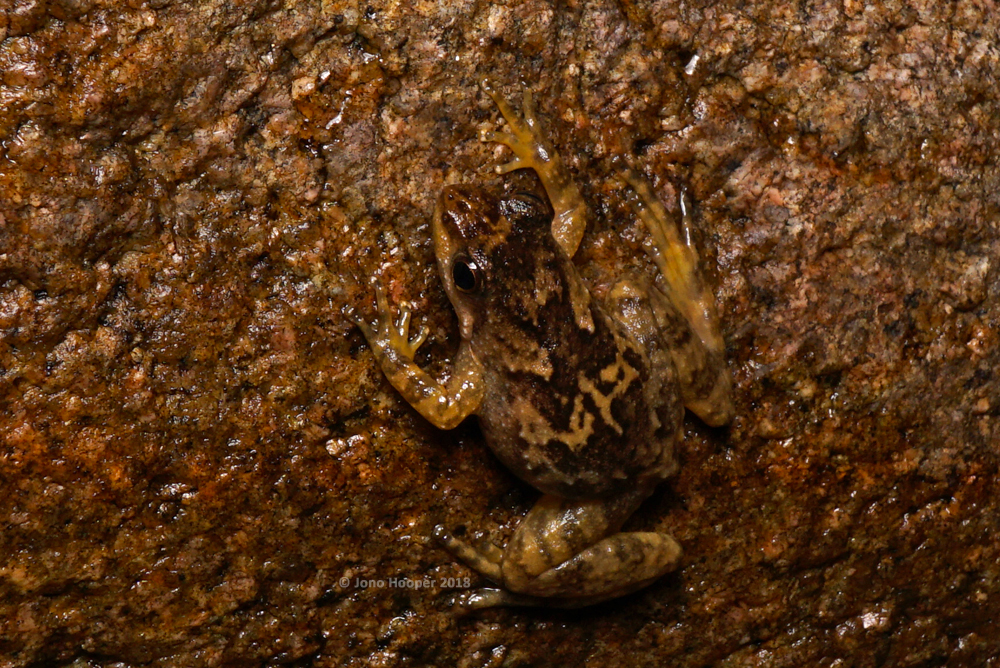This photograph captures a close-up view of a small frog placed prominently in the center, resting on a textured, hard surface that appears to be a rock. The rock itself has a glossy, wet appearance with a predominant rusty orangish-brown hue, interspersed with tan and yellow tones. The frog blends seamlessly into this background with its yellowish-orange body tinged with gray, brown markings, and greenish-yellow legs. The frog's dark brown splotches and yellow and black patterns on its back complement the rock's colors, making the frog almost camouflaged. The frog, which is possibly of the tree frog variety, is facing upward in the image, giving a clear view of its intricate patterns and slightly wet, glossy skin.